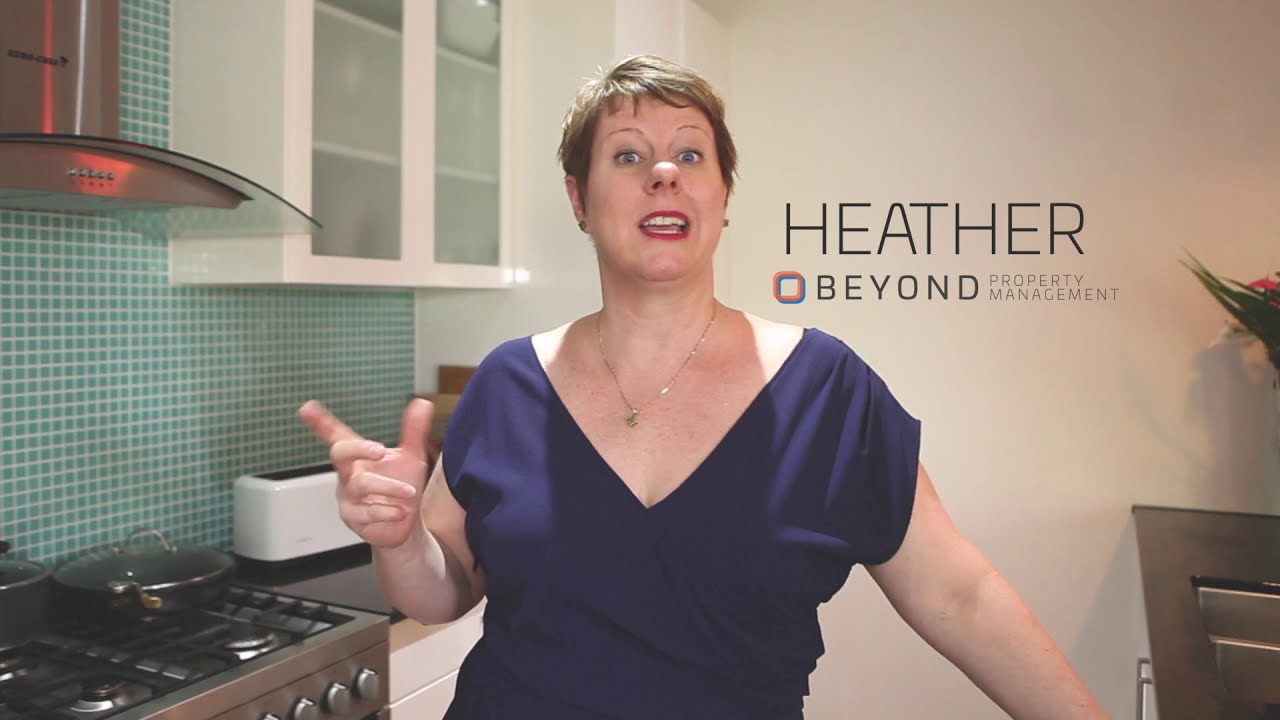The image depicts a middle-aged white woman named Heather, captured mid-presentation in a well-appointed kitchen that appears to be part of an advertisement for her business, Beyond Property Management. Heather, who has short blonde hair and blue eyes, is dressed in a navy blue dress with short sleeves and a V-neckline, accessorized with a gold necklace featuring a pendant and red lipstick. She is animatedly gesturing with her right hand, making a pistol shape as if emphasizing a point. Behind her, the kitchen features a sleek gas stove with a glass range hood, a green mosaic tile backsplash with white grouting, white cabinets, a black marble countertop, and a white toaster. The text "Heather Beyond Property Management" is displayed in black beside her head, indicating her role, presumably as a property manager demonstrating a home or apartment. The scene captures her professionalism and the inviting ambiance of the kitchen space she is showcasing.